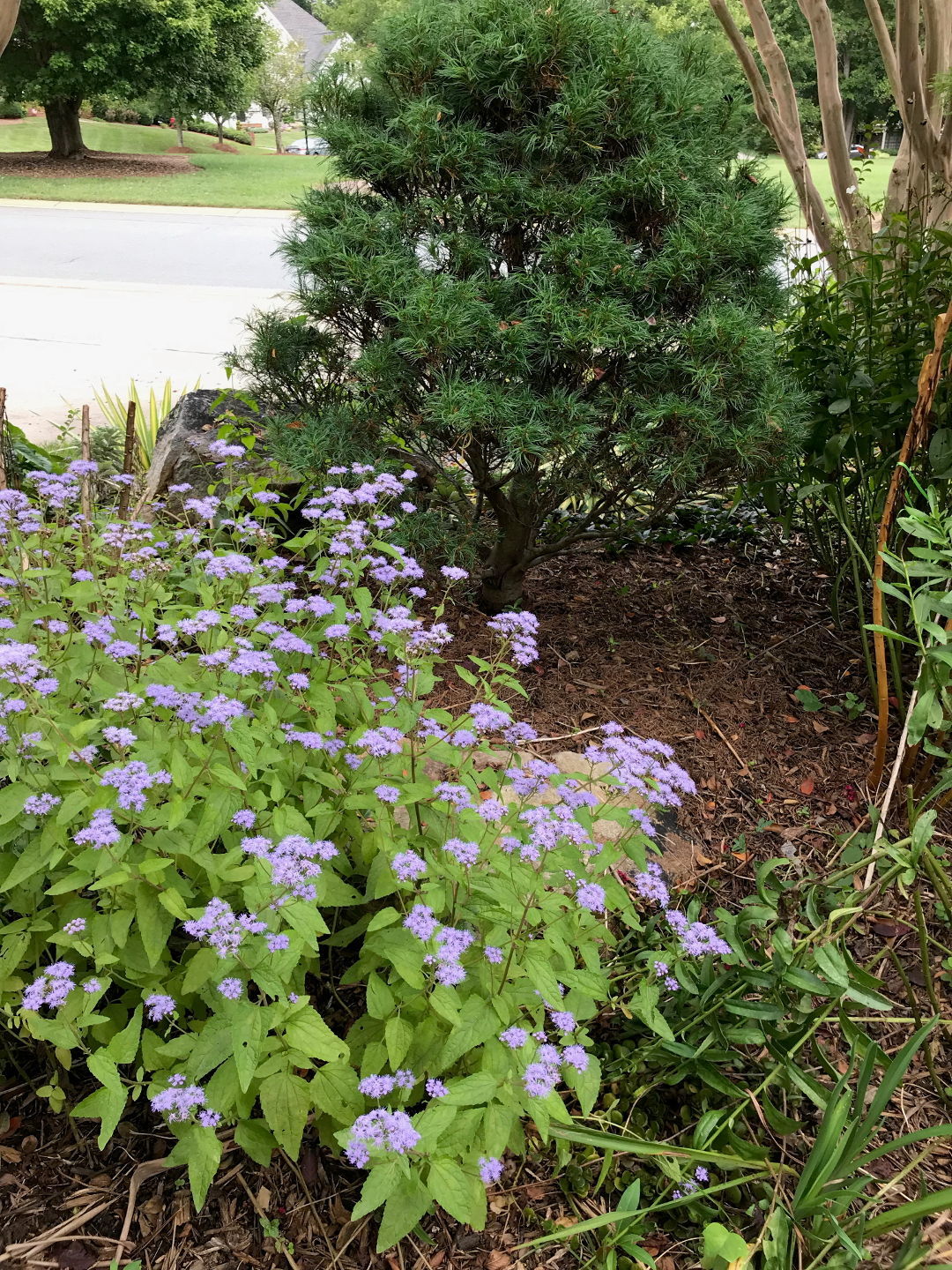In this image, we see a vibrant floral scene centered around a mini tree planted in a bed of brown mulch. In the bottom right-hand corner, dark green blades of grass sprout energetically. To the left of the grass, a plant with light green leaves displays delicate light purple flowers on its slender stems. Dominating the foreground is a tree with robust dark green leaves, while a few brown branches stretch vertically upwards in the top right corner. An orange stake, slightly bent and curving to the right, stands prominently in front of the tree.

On the left side of the image lies a light gray sidewalk, which borders a gray road. Beyond this pathway, a lush field of grass extends, hosting a single tree with deep green foliage. In the distant background, positioned in the top left corner, the gray roof of a house peeks through, adding a subtle sense of depth to the scene.